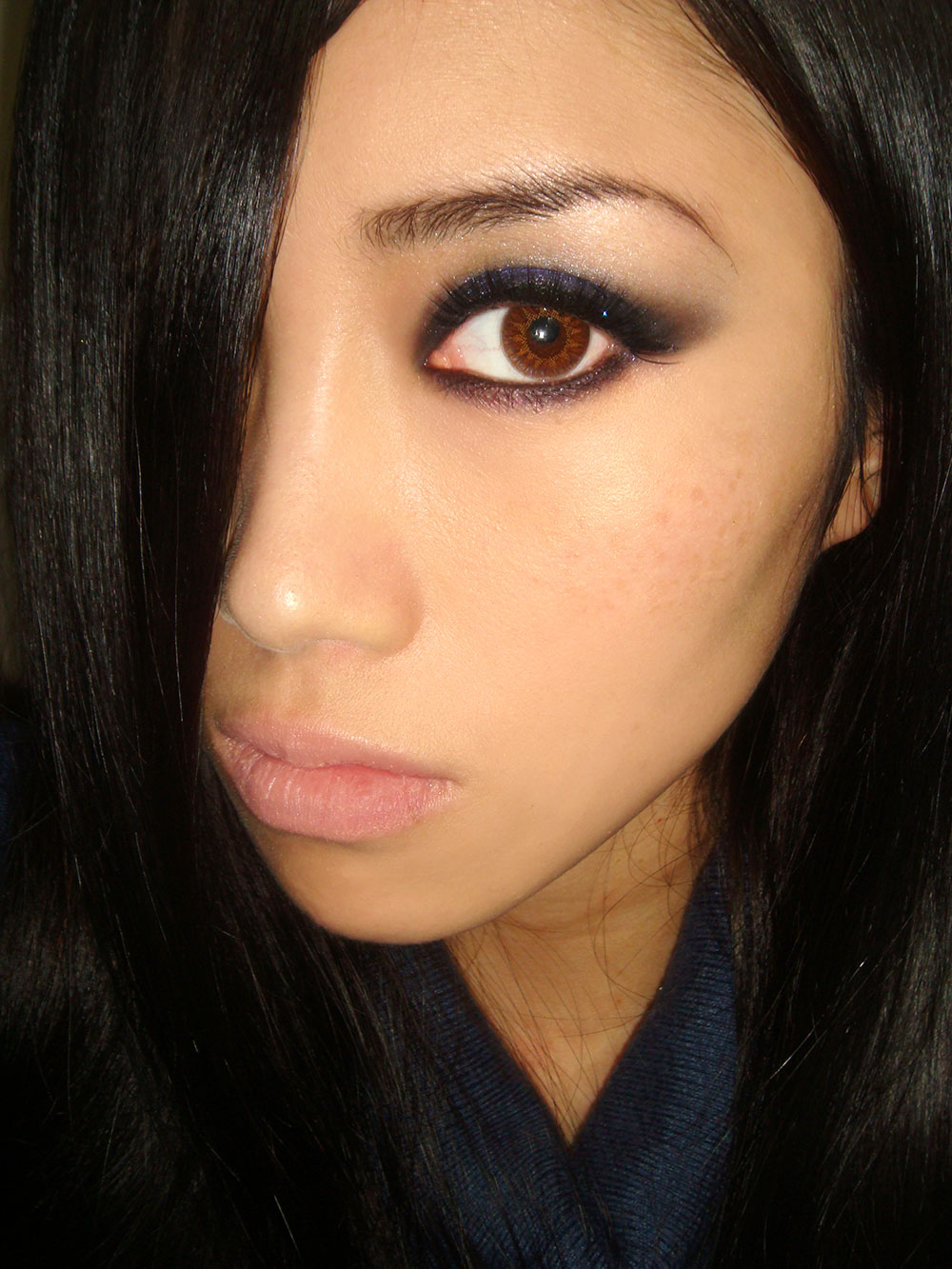This color photograph is a close-up shot of a young woman’s face, likely in her mid-teens, with long, straight black hair that cascades down and obscures her right eye completely. The left side of her face is prominently featured, revealing a brown eye accentuated with mascara and eyeliner, and a blue eyeshadow that adds a hint of color. The reflected light in her pupil suggests she is directly facing the camera. Her pink lips appear without additional color, giving a natural look. She is wearing a dark blue, V-neck top, tight around the neck, that partially frames her face. Her skin tone suggests she is possibly Hispanic. Her head is subtly tilted to the side as she gazes into the camera, with her neatly groomed eyebrows matching the color of her hair.